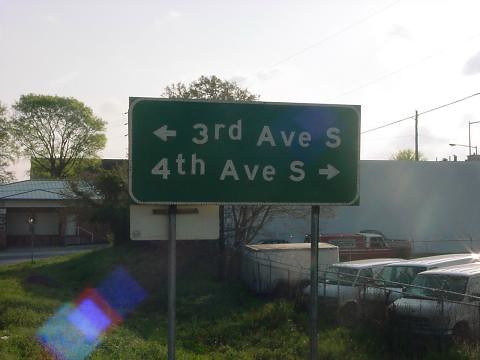The photograph features a rectangular street sign prominently positioned in the center, framed by a rectangular shape with longer top and bottom sides. The green street sign, bordered by a white outline, reads "3rd Avenue S" with an arrow pointing left and "4th Avenue S" with an arrow pointing right, both written in white text. The sign is supported by two silver metal cylindrical poles, each anchored into a grass-covered area. To the right of the sign is a short chain link fence, beyond which several white commercial vehicles are visible, adding a layer of depth to the scene.